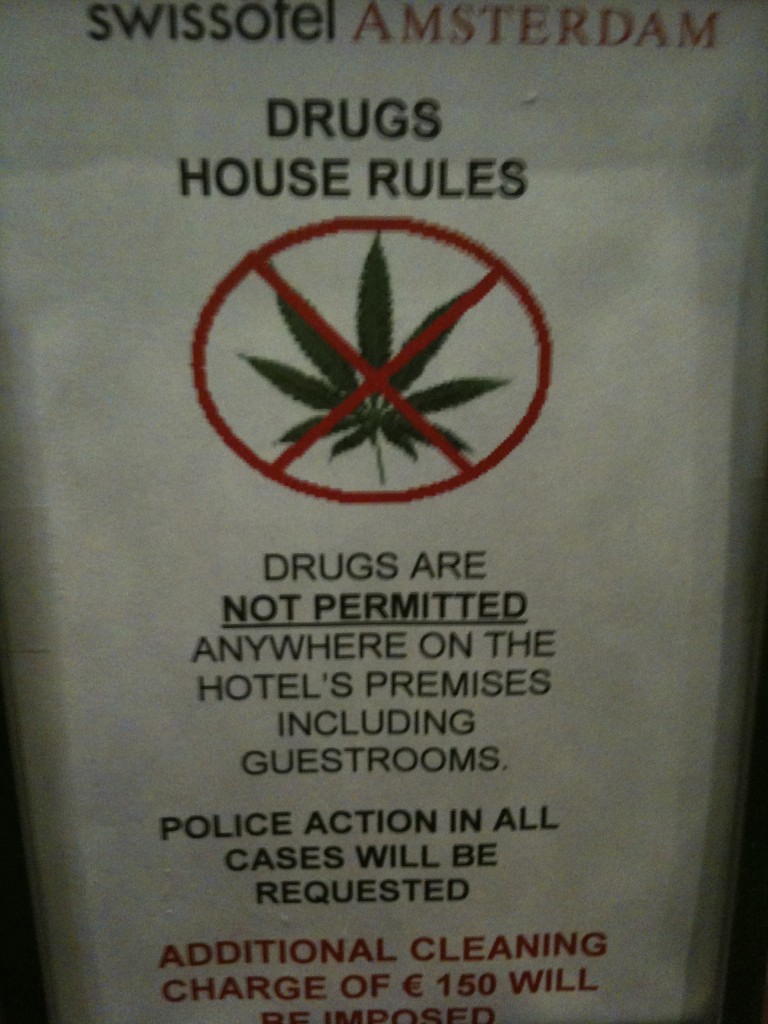This vertical, rectangular image, albeit dark and of low quality, depicts a detailed warning sign posted inside a facility, likely a hotel. The sign, printed on a plain white piece of paper, features both black and red text. At the very top, it states "Swiss Hotel Amsterdam Drug House Rules." Centered below this heading is a prominent green marijuana leaf circled and crossed out in red. Beneath the symbol, a bold and underlined message in black letters reads, "Drugs are not permitted anywhere on the hotel's premises, including guest rooms." Following this, a clear warning in darker black letters mentions, "Police action in all cases will be requested." Lastly, at the bottom in red letters, partially obscured, it indicates, "Additional cleaning charge of 150 pounds/euros will be imposed." The entire image conveys a strict anti-drug policy in a poorly lit environment but remains legible enough to capture all essential details.